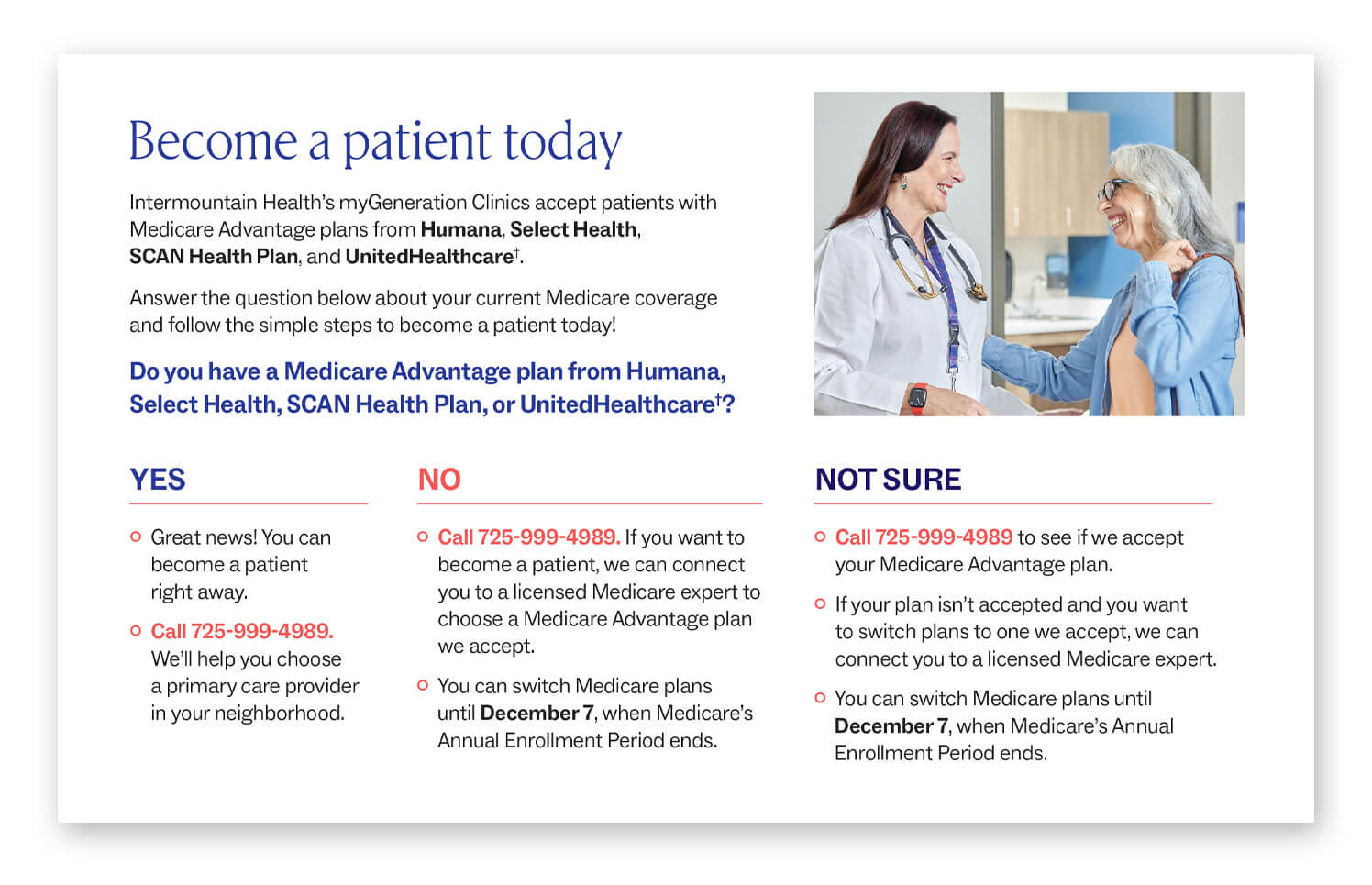**Descriptive Caption:**

The image features a minimalist design with a white square set against a white background. This square contains essential details about becoming a patient at Intermountain Health's My Generation Clinics, which accept patients with Medicare Advantage plans from providers like Humana, Select Health, Scan Health Plan, and UnitedHealthcare. The text invites individuals to answer questions about their current medical coverage and follow simple steps to become a patient. 

For those with an appropriate Medicare Advantage plan, the message encourages them to call 725-999-4989 to start the process and select a primary care provider in their neighborhood. Individuals without a compatible plan or who are unsure about their plan’s acceptance are also urged to call the same number. The message highlights that a licensed Medicare expert can assist in choosing an acceptable Medicare Advantage plan and mentions that Medicare plans can be switched until December 7th, the end of Medicare’s annual enrollment period.